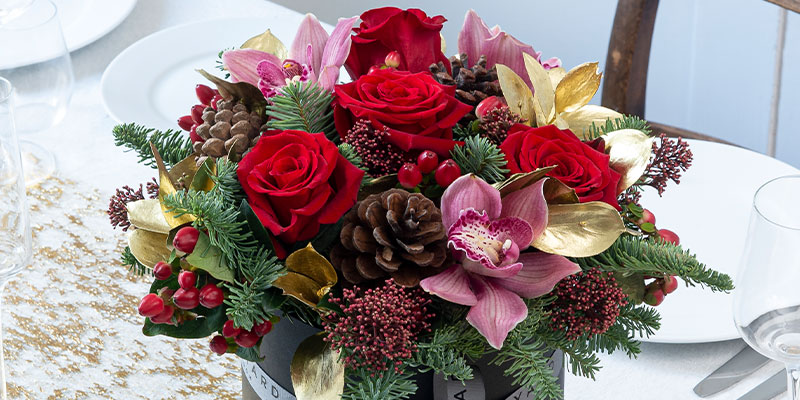This image captures a vibrant and festive floral centerpiece set on a meticulously arranged dining table. The core of the centerpiece features a diverse bouquet comprising four vivid red roses, pink lilies with darker pink spots, and an assortment of sprigs including red holly berries and brown pine cones. Complementing these are green pine needles, yellow leaves, and faux golden leaves, bringing a rich and varied texture to the arrangement. 

The bouquet sits in a black vase adorned with a white label band that partially reads "ARD." The table below is draped in a white tablecloth accented with gold beadwork, enhancing the elegant setting. Surrounding the centerpiece, the table is decked with plain white ceramic plates and transparent wine glasses, indicating readiness for a meal. In the background, the faint shimmer of a brown wooden chair can be observed, adding warmth to the ensemble.

Overall, the bouquet's combination of colorful roses, vibrant lilies, and seasonal elements like pine cones and holly berries, framed by the sophisticated table setting, creates a striking visual indicative of a festive or holiday celebration.